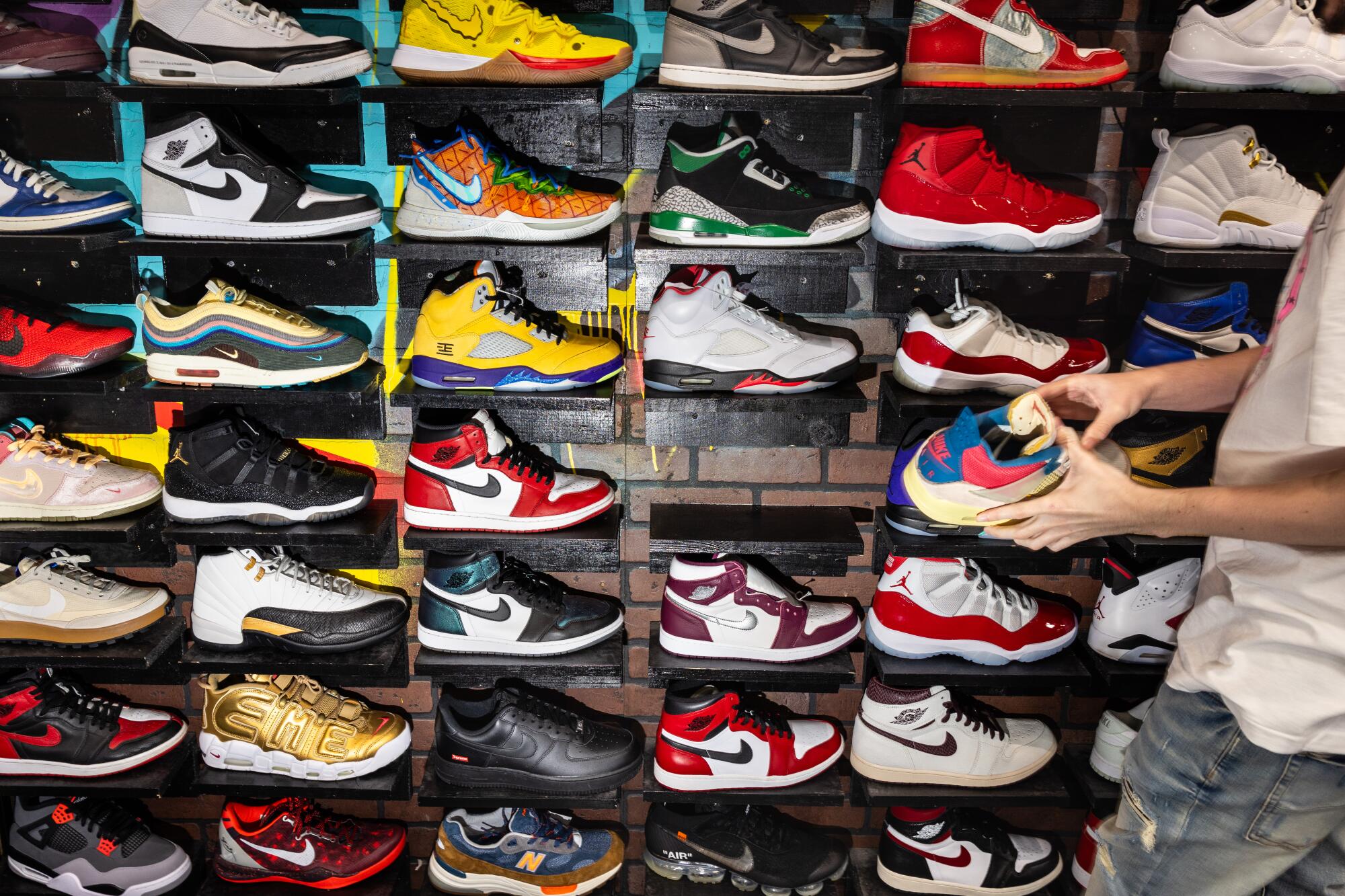The photo showcases a vibrant wall display of over 30 pairs of vintage and collectible Nike shoes, ranging from Jordans to casual dress styles. The shoes come in a myriad of colors including red, yellow, gold, black, white, blue, and gray. They feature various designs such as high-tops, low-tops, Air Maxes, and basketball shoes, all prominently displaying the iconic Nike swoosh. The diverse color palettes include solid colors and combinations like blue and pink. The shoes are meticulously arranged on shelves mounted to what appears to be a brick or brick-like wall. On the far right of the image, a person is partially visible, wearing a white t-shirt and distressed blue jeans. His hands, which are a medium skin tone, are seen reaching for a closer inspection of a blue and pink shoe, embodying the interactive and engaging atmosphere of the urban-style shoe store, possibly akin to a Footlocker.